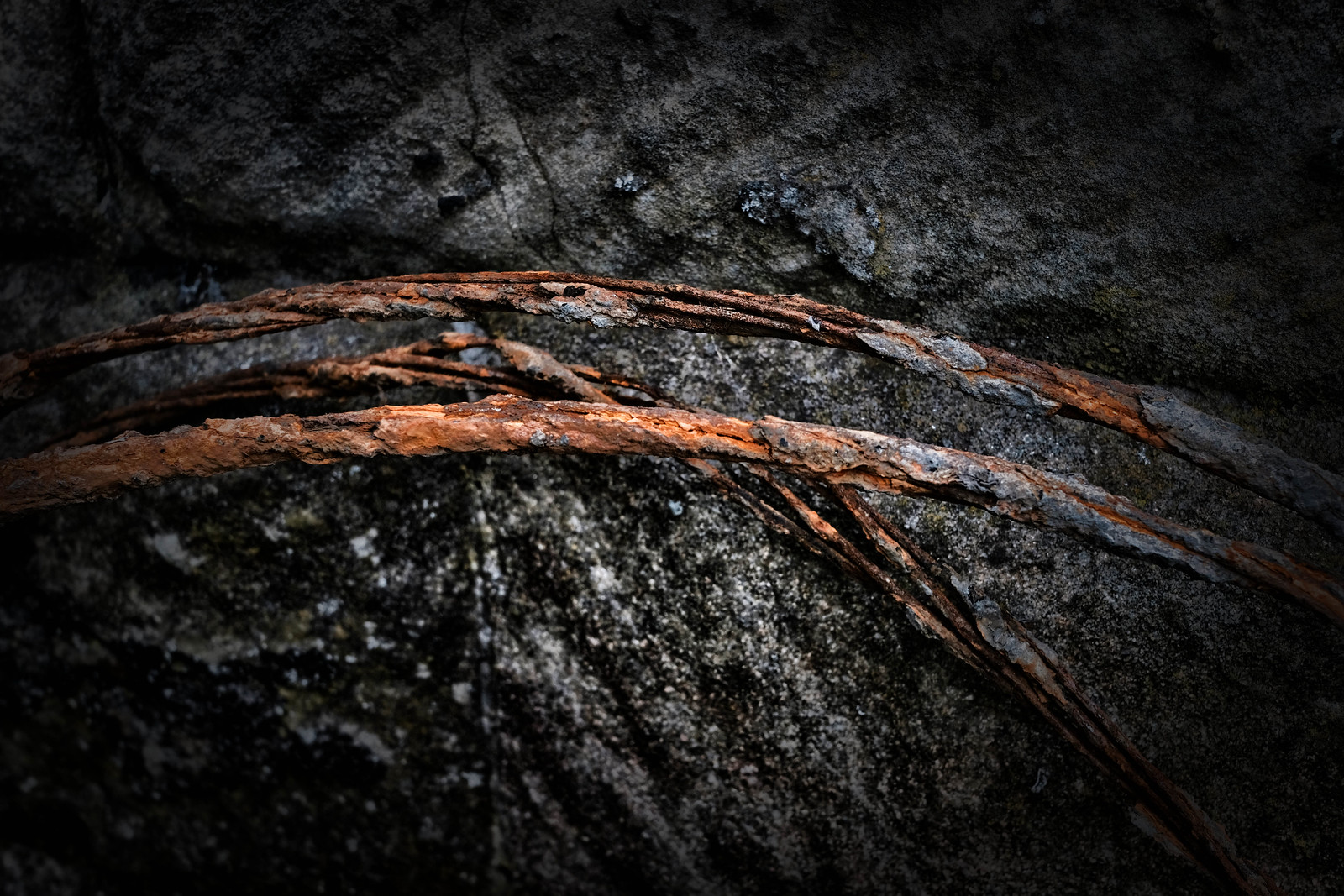This image captures a close-up of what appears to be three brown, twisted objects resembling tree branches or possibly rusted metal cables, set against a predominantly black and rough-textured surface. The black surface, which some might interpret as sticky tar or rough black rock, features uneven lighted patches making certain areas look white. The edges of the image are darker, with the rough texture extending outward. The branches or cables form distinct shapes, with two nearly parallel and the third diverging downward towards the lower right corner, creating a dynamic composition. Scattered white and green splotches add to the gritty, weathered appearance, enhancing the contrast between the organic-looking branches and the harsh, textured background.